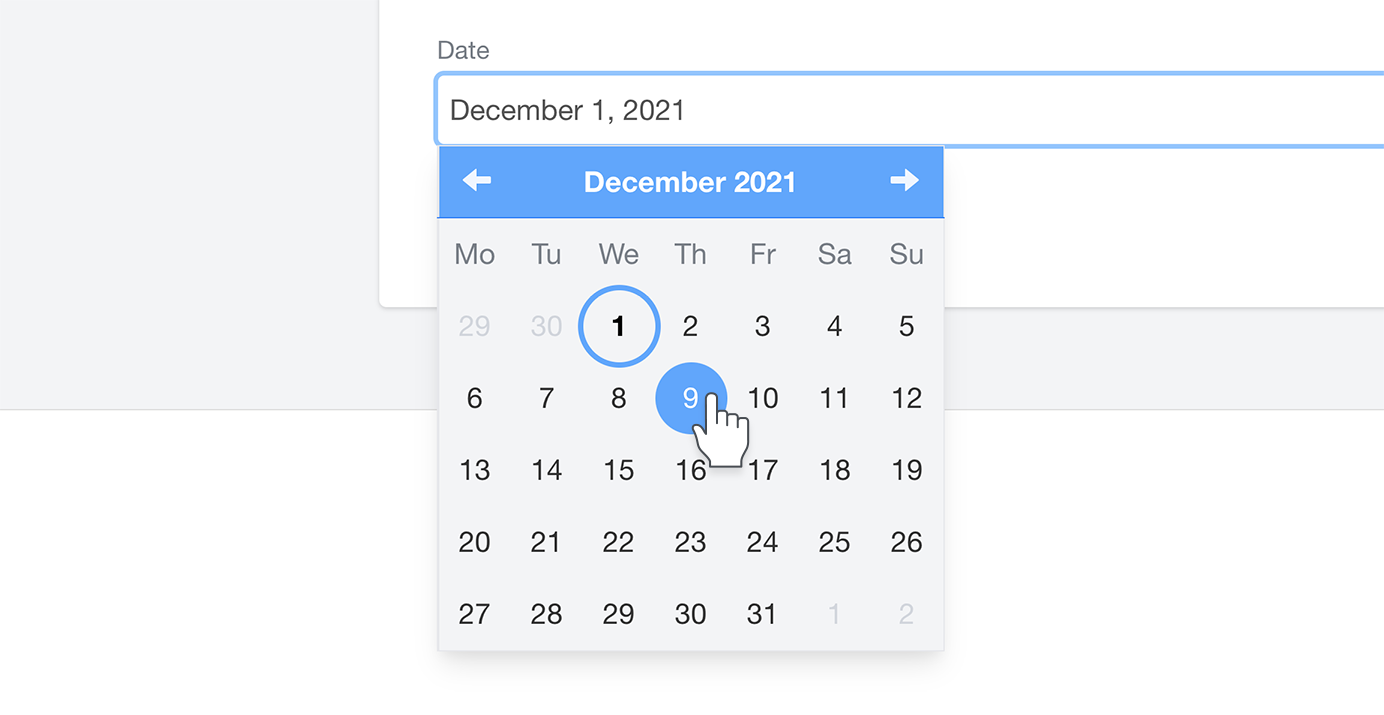The image depicts a date selection interface on a web page for December 2021. The current date displayed is Wednesday, December 1st, 2021, highlighted in a white text field. The interface shows a calendar grid, where the selected date has a blue circle outline, indicating it is not the active choice. The date "9th" is prominently highlighted with a solid blue fill, showing a cursor hovering over it, suggesting the user intends to change the selected date from the 1st to the 9th. The overall design is characterized by a clean white box containing the date elements, set against a gray background, indicating a simple and straightforward date selection process. The image appears to be a section of a larger web page interface.